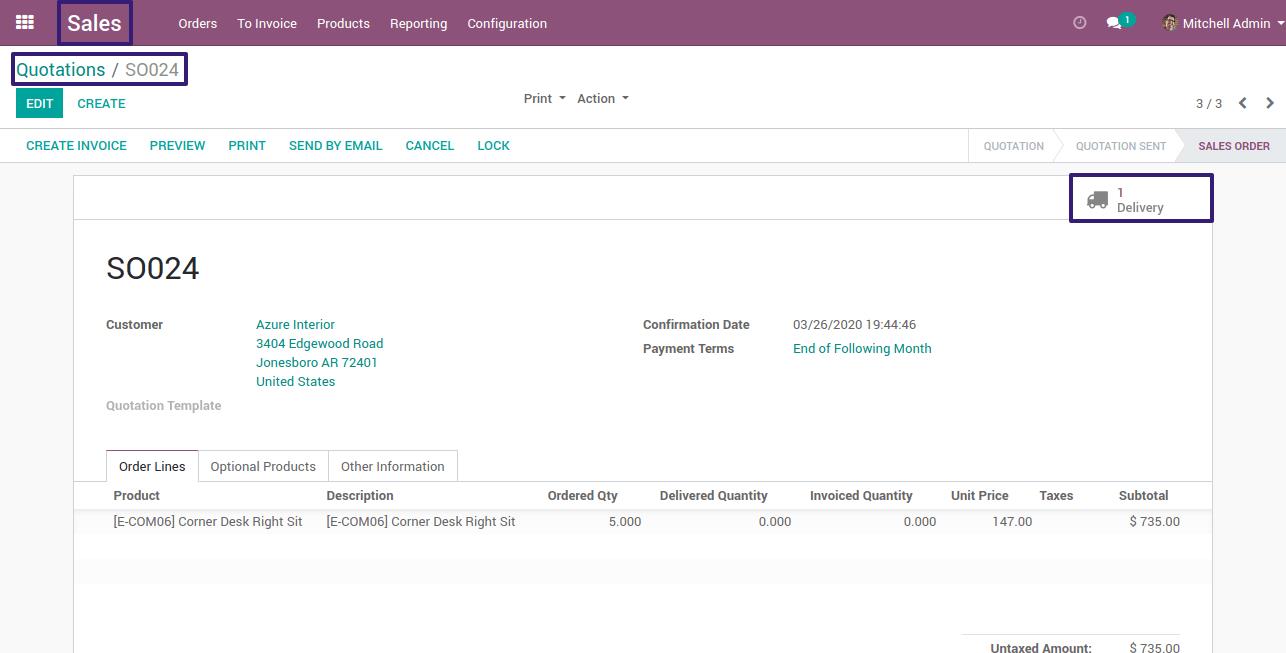The image captures a screenshot from a computer screen displaying a sales management interface. At the top of the screen, a header section is presented in a rose-colored, almost purplish hue, enclosing a navigation bar. On the left, there is a cube icon made up of nine smaller squares, indicating the main menu, followed by the word "Sales" in white text, itself encapsulated in a navy blue rectangle.

Moving rightwards across the navigation bar, you find white text links labeled "Orders," "To Invoice," "Products," "Reporting," and "Configuration." Beside these links, there are additional icons and text: a tiny clock icon, two speech bubbles with a green circle containing the number one, and the user's name displayed as "Mitchell Admin."

Beneath the header, in teal print, the text "Quotations / SO-0024" is visible. Following this downward, another row of options includes "Edit," "Create," "Create Invoice," "Preview," "Print," "Send by Email," "Cancel," and "Lock."

Towards the lower part of the screenshot, there is a section highlighted by a blackish-purple rectangle featuring a truck icon with a number one, indicating the delivery status.

This descriptive caption provides a detailed walkthrough of the screenshot elements, ensuring comprehensive clarity.